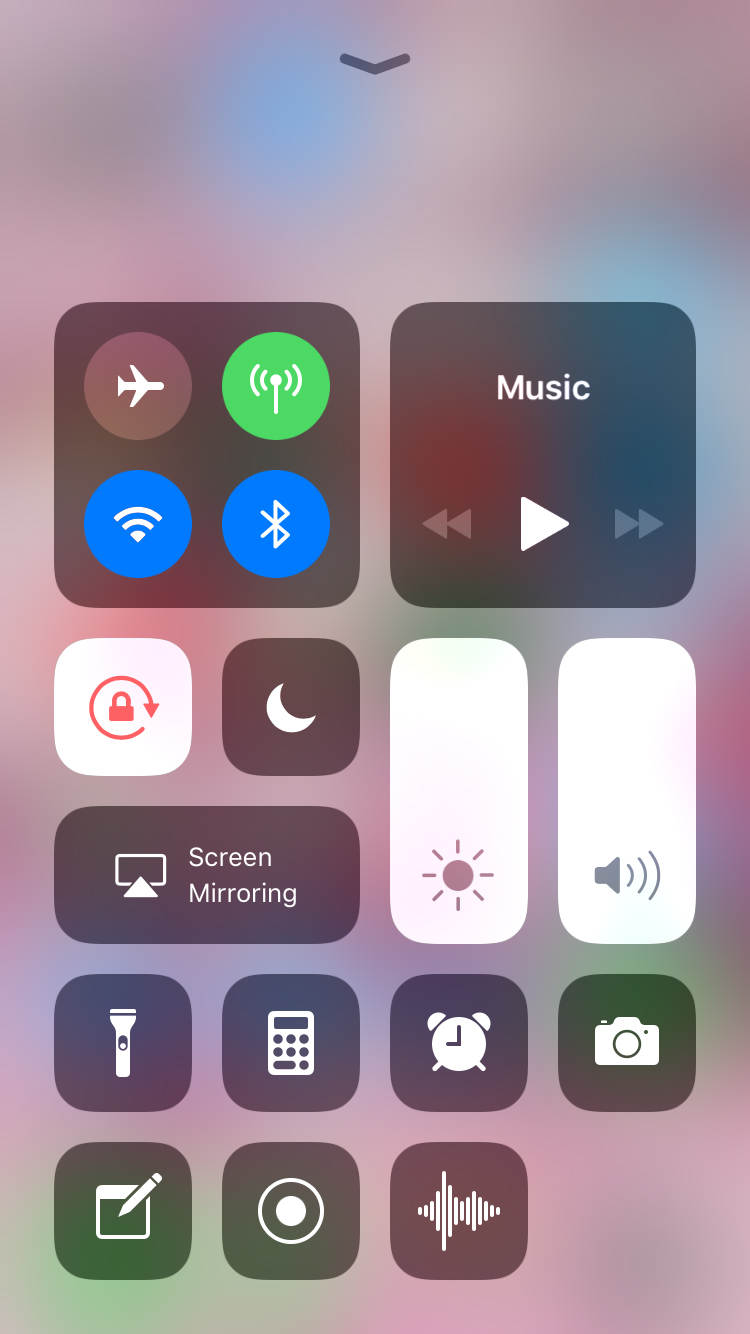The image displays a smartphone screen featuring numerous functional options organized into panels. The main feature includes two prominent brown-colored panels, each serving different purposes. 

The first brown panel, positioned on the left, showcases four circular icons arranged vertically: 
1. A brown circle with a white airplane symbol, likely indicating Airplane Mode.
2. A green circle emitting radar-like signals, which could represent a GPS or radar function.
3. A blue circle depicting Wi-Fi signal strength.
4. A blue circle with a Bluetooth icon.

Adjacent to it, the second brown panel simply reads "Music" in white text at its center. Below this text, there are playback controls: a play button flanked by rewind and fast-forward buttons on either side.

Beneath these prominent panels, there is a series of smaller panels:
1. A panel with a lock icon and a red arrow around it, possibly indicating a rotation lock function.
2. A brown panel with a crescent moon symbol, probably signifying Do Not Disturb mode.
3. Another brown panel with an icon for screen mirroring.
4. A white vertical panel with a light bulb emitting rays, likely representing a brightness toggle or flashlight function.
5. A panel with a speaker icon, which might control sound settings.

Following these, there are seven additional small brown rectangles, each containing different icons:
1. A torch, representing the flashlight function.
2. A calculator icon.
3. An alarm clock.
4. A camera.
5. A notepad.
6. An icon that appears to be a circle within a circle, which is ambiguous.
7. An icon that resembles a speech recorder, possibly for voice memo recordings.

The overall layout is meticulously organized, providing quick access to an array of controls and applications.